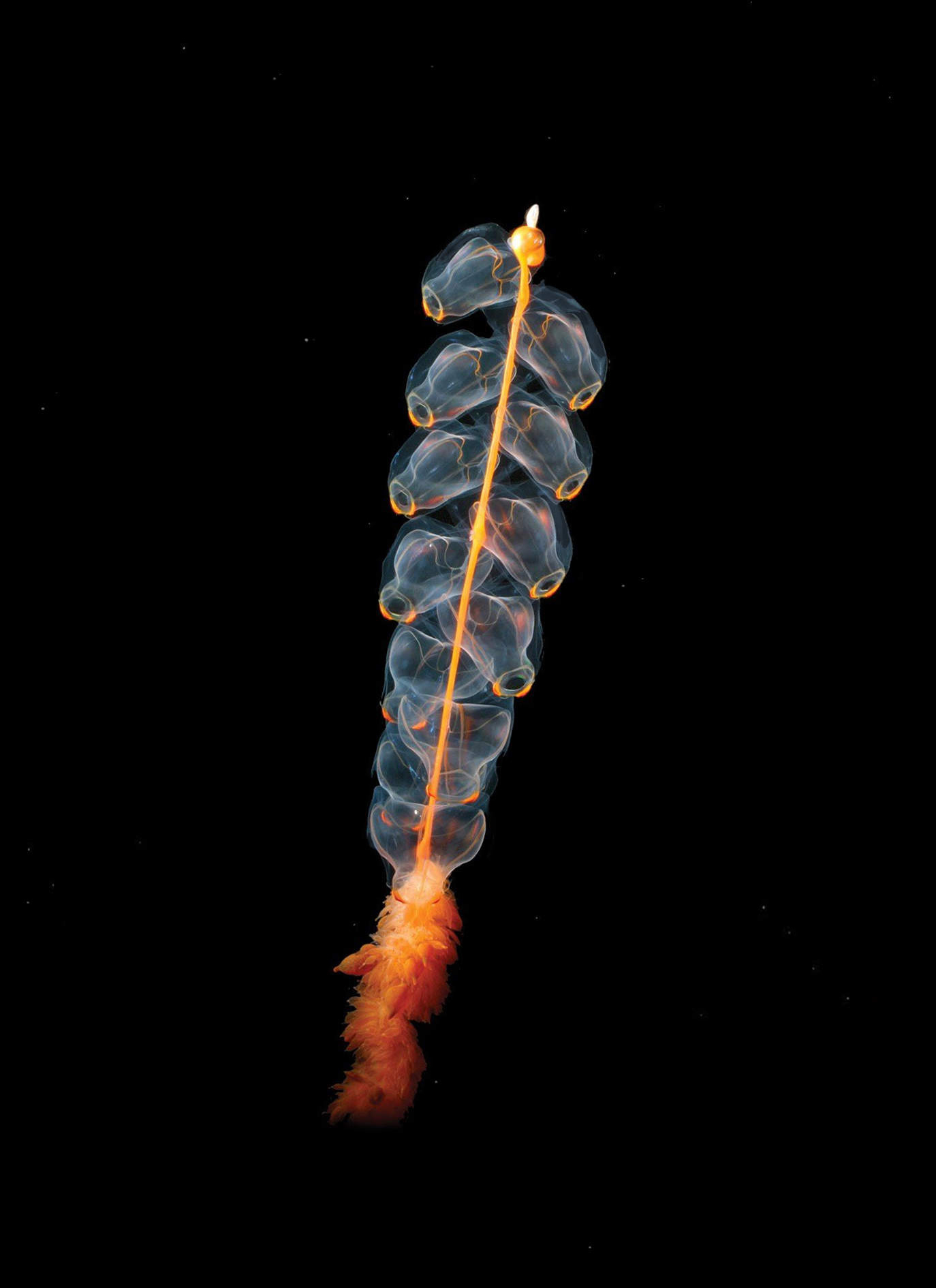The image depicts a peculiar underwater organism that appears to blur the lines between aquatic plant and creature. Emerging from a fuzzy, vibrant orange base, an equally orange stem rises gracefully to the midpoint of the composition. The stem, resembling a spine if viewed as an animal, supports an array of translucent appendages – about ten on each side. These appendages extend outward and feature subtle bluish-gray hues accentuated by orange tips. The entire scene is set against a stark black background, which dramatically showcases the intricate details and vivid colors of the specimen, highlighting its enigmatic and otherworldly beauty.